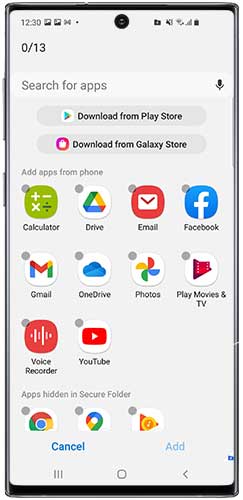Screenshot of a smartphone's app management screen:

In the upper left-hand corner of the screen, black text displays the time, accompanied by several icons such as the battery indicator on the far right and a network connection signal strength meter to its immediate left. Additional icons are present but unclear in their function. Below this status bar, on the left side, black text reads "0-13." To its right is a search box featuring gray text that prompts the user to "Search for apps," with a small microphone icon for voice input.

The interface includes two prominent buttons beneath the search box: "Download from Play Store" and "Download from Galaxy Store." Further down, the text "Add apps from phone" appears above a list of app icons arranged in three rows. The first row includes: a calculator, Google Drive, and email. The second row features: Facebook, Gmail, and OneDrive. The final row includes: Google Photos, Play Movies, a voice recorder app, and YouTube.

Moving further down, the section "Apps hidden in Secure Folder" displays three icons, with one identified as Chrome while the other two are not clearly discernible. At the very bottom of the screen, two buttons, "Cancel" and "Add," allow the user to finalize their app selection actions.